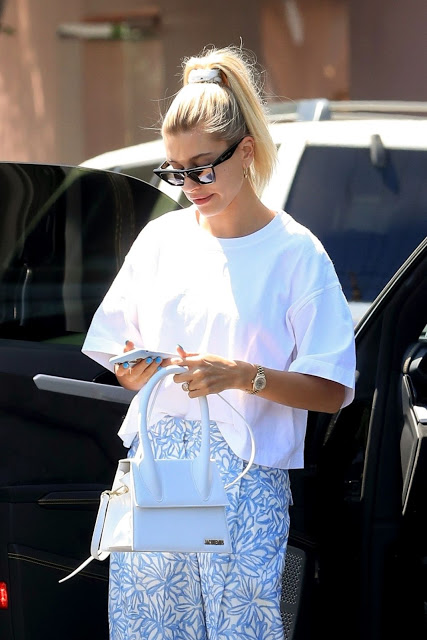The photograph captures a blonde woman standing outside a black car with its door open, revealing a tinted window and black interior. Behind her, there's a white SUV and a brown wall. The main focus is on the woman, who exudes a casual yet elegant style. She wears a loose, baggy white short-sleeve t-shirt paired with white pants adorned with light blue floral embroidery, giving off a high-quality, summer-fashion vibe. Her accessories include a white purse from Jack Kemmer, a silver watch on her left wrist, and a large ring on one of her fingers. She holds a white smartphone in her right hand while gripping the purse's strap. Her blonde hair, darker at the roots, is styled in a high ponytail secured with a white scrunchie. She also sports stylish sunglasses with dark frames and transitioning lenses, gold earrings, and baby blue manicured nails. The overall scene suggests she might be in the midst of a casual outing, accentuated by the blend of elegance and relaxation in her attire.